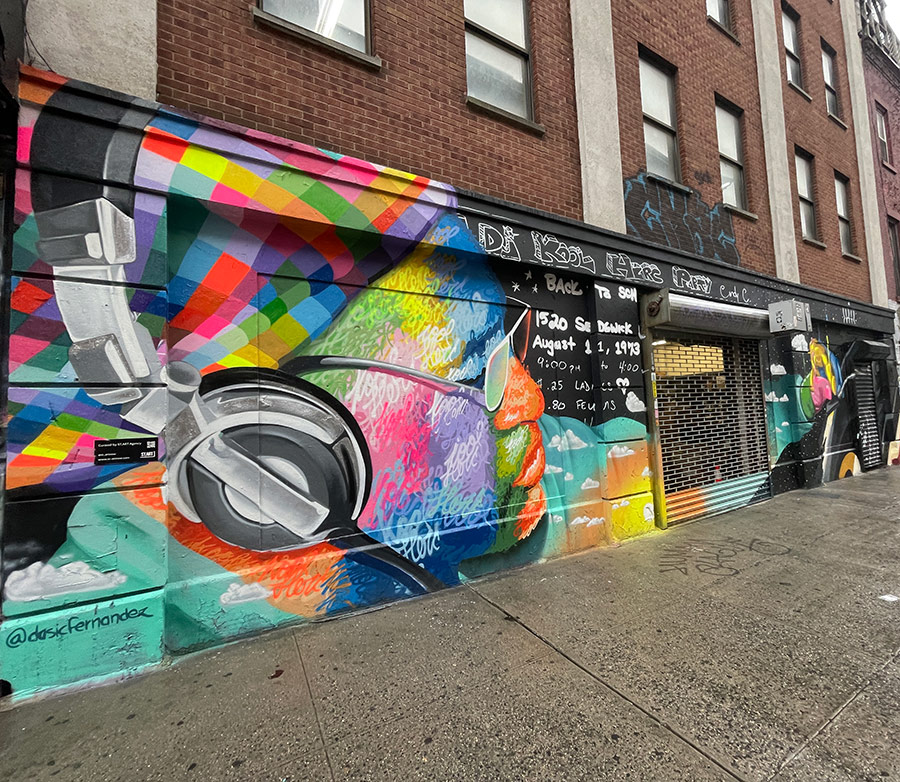The photograph captures a vibrant city street scene, with a detailed mural painted on a stone and brick wall of a building. The mural, signed by the artist Dasic Fernandez, features a photorealistic depiction of a man with closed eyes, wearing silver headphones, glasses, and a rainbow-colored knit hat or do-rag. His face and shoulders are composed of bright, multicolored squiggled lines, adding an intense and lively visual effect. Additionally, there are small white clouds painted in front of his body. The mural contains the text "1520" and "August 11, 1973."

The bottom portion of the building includes access doors for vehicles and pedestrians, covered with graffiti, and gated open doorways to the right. The top half of the building showcases red brick and concrete columns, segmenting it into three sections adorned with windows. There's a hint of blue graffiti underneath the central part of the windows. The sidewalk in front of the building is made of worn concrete with exposed aggregate, tar patches, and graffiti markings. Adjacent to the mural, another part of the building is painted black with red-brick extensions above it. The overall scene is a vivid, colorful testament to urban artistry and city life.